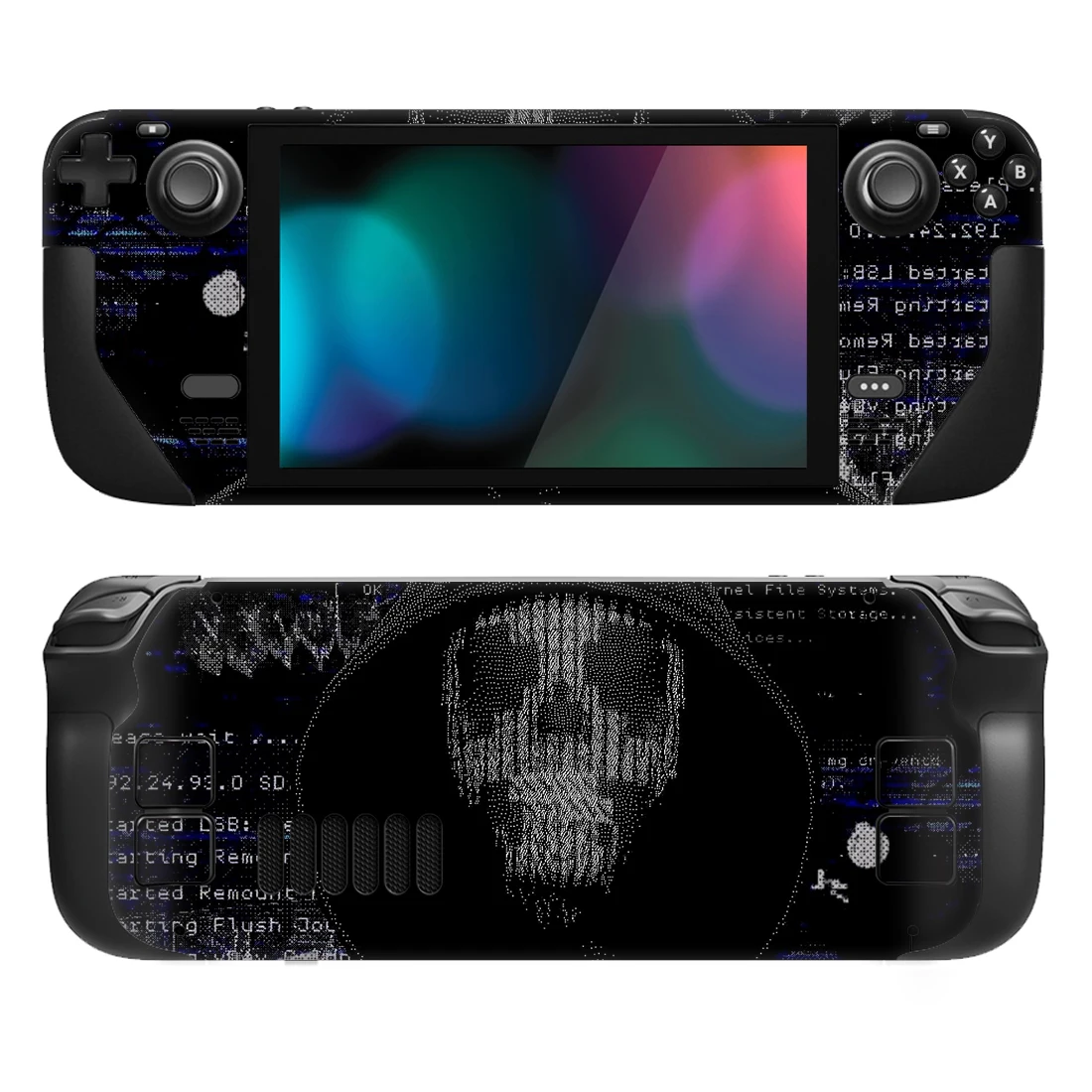The image features two photographic views of a sleek, black rectangular gadget with curved corners, resembling a combination of a radio tuner and a game controller. The device is displayed on a white background. The front view of the device showcases a central LCD screen adorned with gradient blue and pink circles, flanked by two knobs on either side. The screen displays backward text that spells out "REMOL8BV."

Adjacent to the knobs, there are additional buttons suggesting interactive functionality, reminiscent of a game controller setup. The overall theme of the gadget leans heavily towards technological utility, possibly a specialized controller or tuner.

The back view highlights a curved black surface dominated by a graphic of a skull wearing a hoodie, rendered in shades of gray and dark gray. Surrounding the skull, white text reads "92.24.98.0 SD," along with additional character sequences including "Rated DSB," "Rating REM," and "RTING flush JOL." Another notable detail includes the appearance of the word "RENCO" potentially marking a brand name. A round, whitish object, likened to an old-fashioned bomb, is partially visible towards the bottom right of the backside image, adding an intriguing element to the design.